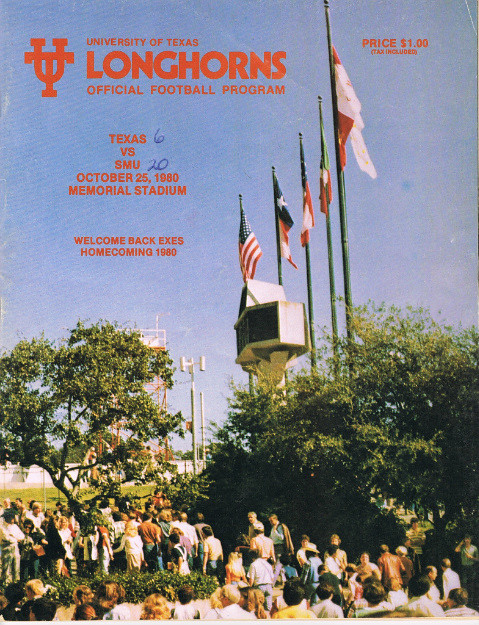This vertically aligned rectangular image is the front cover of an aged football program or magazine, highlighting a special event. The color scheme includes light blue, red, white, black, green, gray, orange, yellow, and brown. The top section features a blue sky backdrop and text in red, indicating a price of $1, tax included, positioned in the upper right corner. To the left, it reads "University of Texas Longhorns" with the Longhorns logo, followed by "Official Football Program" underneath. In the center of the cover, it prominently states "Texas vs. SMU, October 25, 1980, Memorial Stadium," with an annotation in blue ink noting the final score as "Texas, 6 - SMU, 20." Below this, there's a welcoming note for Homecoming 1980 with the phrase "Welcome Back X's."

The middle portion of the image displays several flags on poles, including the American flag, the Texas flag, and three others, against the blue sky. Trees lined up near the bottom frame the setting, where a large crowd of people is seen walking towards or entering the stadium, imparting a vibrant pre-game atmosphere. This cover captures the essence of a historic football event at the University of Texas, held at Memorial Stadium.